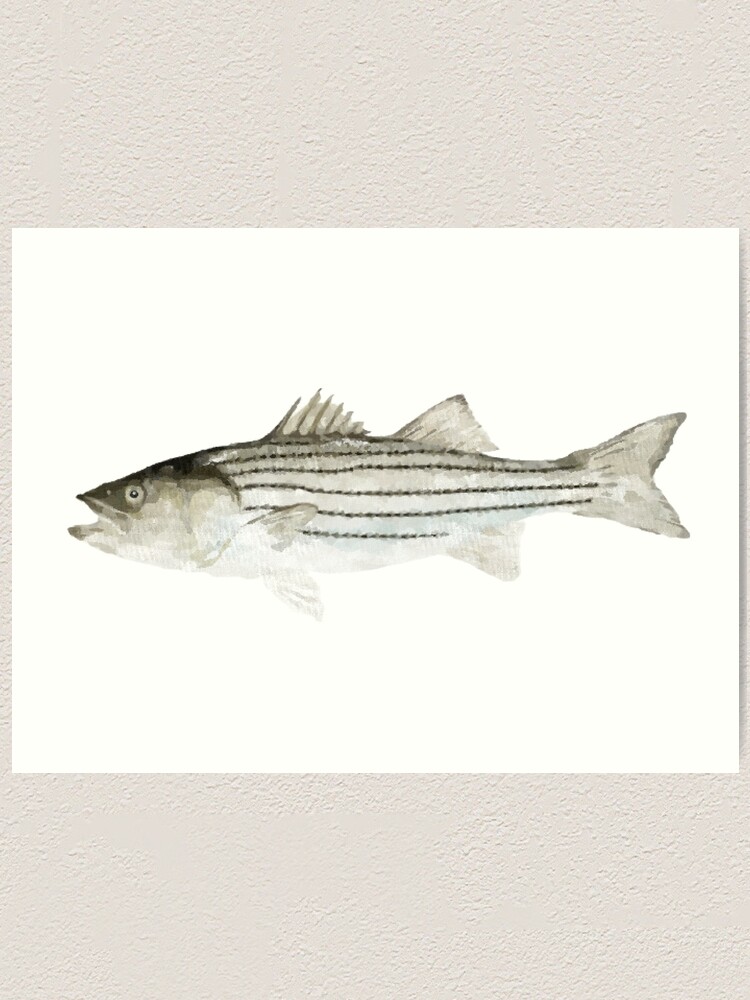The image depicts a traditional fish illustration, most likely a watercolor drawing on white paper, set against a gray or off-white background. The fish, which is shown in profile and facing left, displays a remarkable level of detail and craftsmanship. It is primarily rendered in grayscale, with subtle blue accents beneath the lower gills to add a touch of three-dimensionality. The fish has its mouth open and one eye visible, which appears to be looking at the viewer. Horizontal black stripes run lengthwise along its body. The fish also features multiple fins: two at the front, one on the back of the belly, a tail at the rear, and two fins on its back. The overall image appears to be a photograph of this finely executed fish illustration.